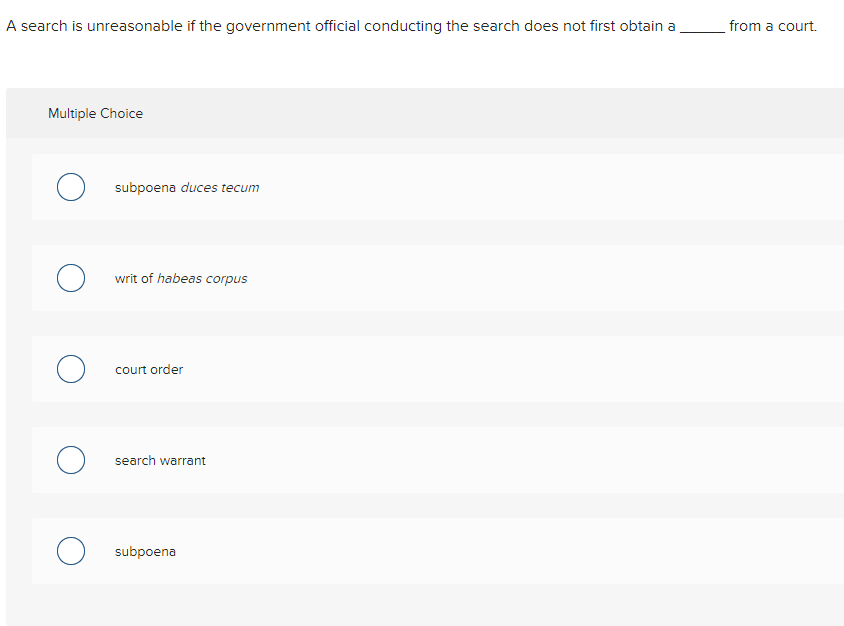This is a detailed descriptive caption for a quiz question screenshot:

---

The image showcases a screenshot set against a white background. At the top of the image, a query is presented in black text: "A search is unreasonable if the government official conducting the search does not first obtain a ____ from a court." The blank is emphasized with an underscored black line, indicating the missing term.

Beneath the question, there is a multiple-choice format displayed within a gray box. The top segment of this box, darker gray in color, is labeled "Multiple Choice" in black text.

The options for the question are listed below this header in individual light gray boxes. Each option is associated with a white or black font and is situated inside its respective compartment, which features a slightly darker gray top border. Each choice also has a round circle to its left, unselected in blue, serving as a selection option indicator.

The five choices provided are:
1. Sapona Dukas Tikam
2. Writ of Habeas Corpus
3. A Court Order
4. A Search Warrant
5. A Subpoena

Each option box has light gray padding above, below, and to the left, providing clear delineation from one another, while the right side lacks additional padding, keeping the design compact.

Overall, the layout is clean and structured, designed to facilitate ease of reading and selection in a multiple-choice format.

---